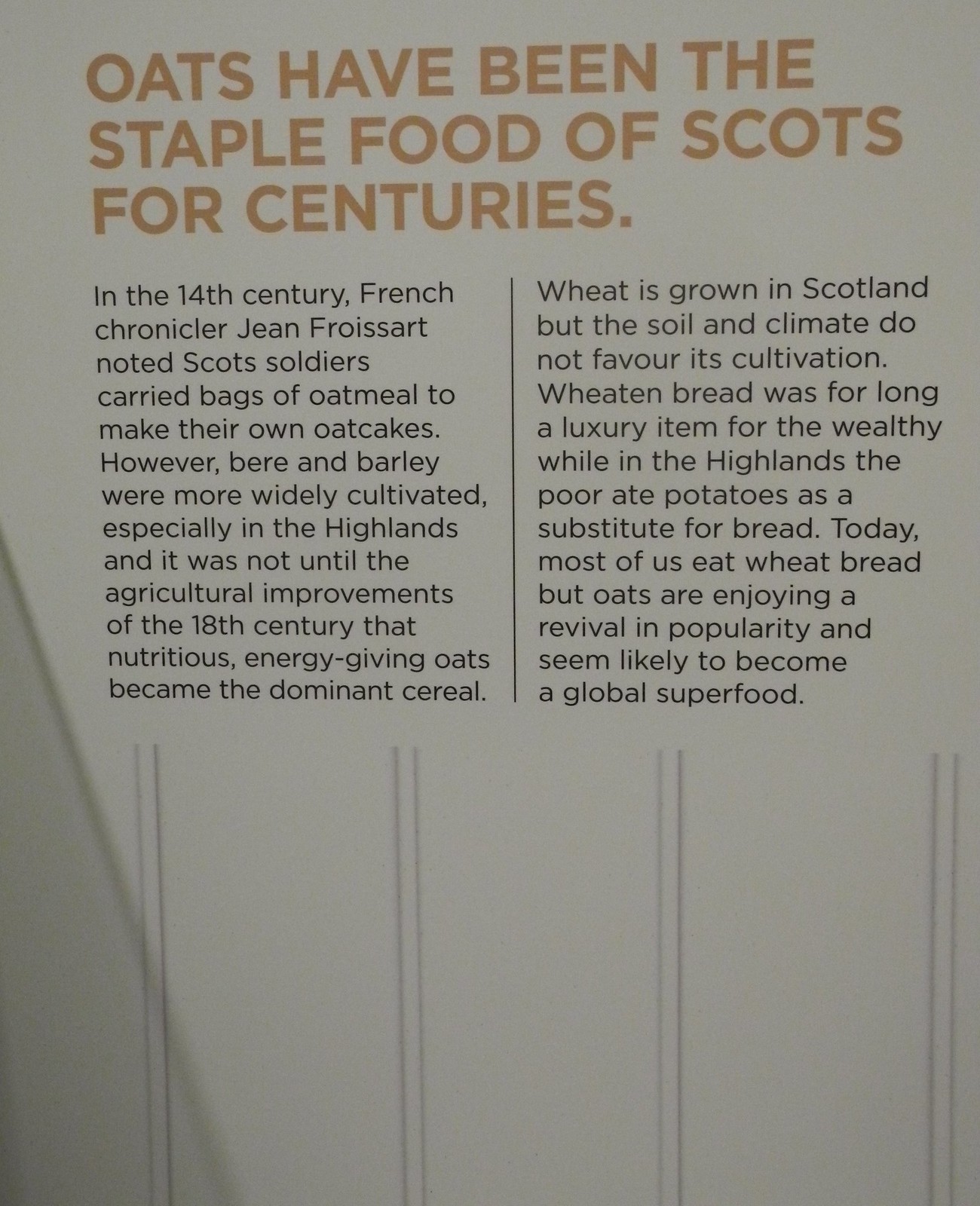The image is a color photograph in portrait orientation, featuring an informational poster at the upper half. The poster is predominantly white with a golden yellow-brown heading in all capital letters that reads, "OATS HAVE BEEN THE STAPLE FOOD OF SCOTS FOR CENTURIES." Below the heading, the text is divided into two columns separated by a vertical black line. The content begins with an account stating that in the 14th century, French chronicler Jean Frassart noted Scots soldiers carried bags of oatmeal to make their own oat cakes. The text elaborates that barley and bear were more widely cultivated, particularly in the Highlands. It was only with the agricultural advancements of the 18th century that oats became the predominant cereal, recognized for their nutritious and energy-giving properties. The narrative continues to explain that wheat, although grown in Scotland, was not favored due to unsuitable soil and climate, making wheat bread a luxury item for the wealthy. In contrast, the poorer populations in the Highlands typically ate potatoes instead of bread. Today, while wheat bread is common, oats are experiencing a resurgence in popularity and are poised to become a global superfood. The overall photographic style of the image is realistic, capturing the detailed text and the white panel board with vertical stripes visible near the bottom.